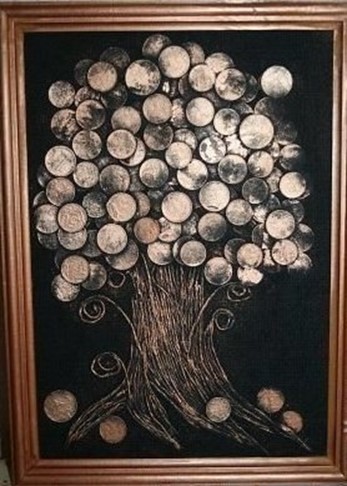The image features a vertically oriented, dark artwork set against a black background, housed in a wooden frame with a coppery-gold hue. Dominating the scene is a meticulously crafted tree made from silver coins, some of which have been artistically oxidized to display varying shades from black to copper. These coins form the leaves densely clustered together. The tree's trunk and branches are intricately shaped from thin lines of copper wire, which converge into a detailed root system at the base. Scattered coins at the bottom give the impression of fallen leaves, adding a touch of realism to this unique metal art. The overall color scheme of the tree includes brown, cream, and white tones, creating an evocative and tactile visual experience.